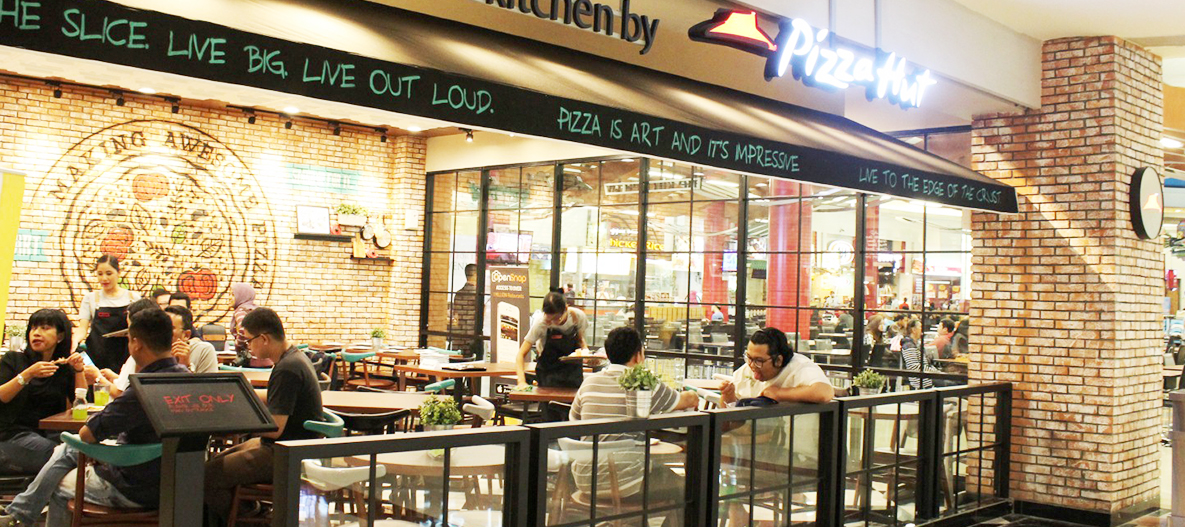The image captures a bustling scene at an outdoor patio of a Pizza Hut restaurant, showcasing a blend of modern and inviting ambiance. Dominating the top right of the photograph is a prominent neon sign with the Pizza Hut logo, illuminated in bright white. Beneath this, stretching across a canopy, is the slogan "Live Big. Live Out Loud. Pizza is Art and It's Impressive." Below, a vibrant atmosphere unfolds with a mixture of dining tables and chairs, where numerous patrons are seen eating and engaging in conversations. The open-air setting includes waitresses attending to customers, enhancing the lively scene. The background features a brick wall adorned with various fabric patterns and a notable circular painting, adding a splash of artistry to the space. Amidst the diners, a red sign indicating "Exit Only" is visible. The overall composition suggests a realistic and representational style, possibly situated in a mall or airport, offering a vivid snapshot of communal dining at Pizza Hut.